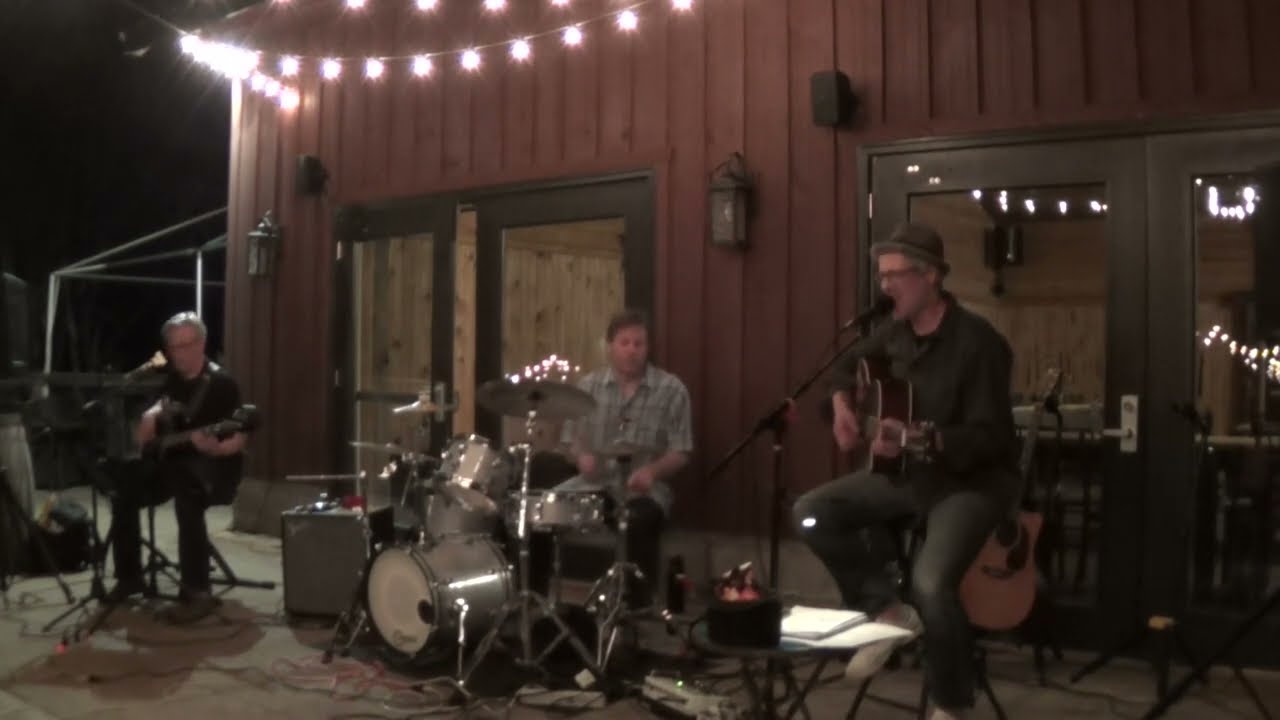Outside a building with vertical reddish-brown wooden paneling and green-framed doors, a three-man band performs under the night sky, illuminated by strings of multicolored lights draped above. The setting appears to be a patio, suggesting a casual, possibly bar-like venue. Each doorway, including a glass one on the left, frames the scene. The lead singer, a tall man around 40 wearing a gray cap perched loosely on his head, strums an acoustic guitar while singing into a black standing microphone. In front of him, a circular table holds a white book. The bassist, situated on the left, sports an all-black outfit and gray hair, contrasting with his acoustic guitar. In the middle, the drummer, dressed in a gray plaid shirt and black pants, keeps the rhythm on his drum set. The scene features additional musical gear like amplifiers and an extra guitar positioned behind the singer. The atmosphere conveys a mellow, possibly alternative or country music vibe, with no visible patrons and an open sky above.